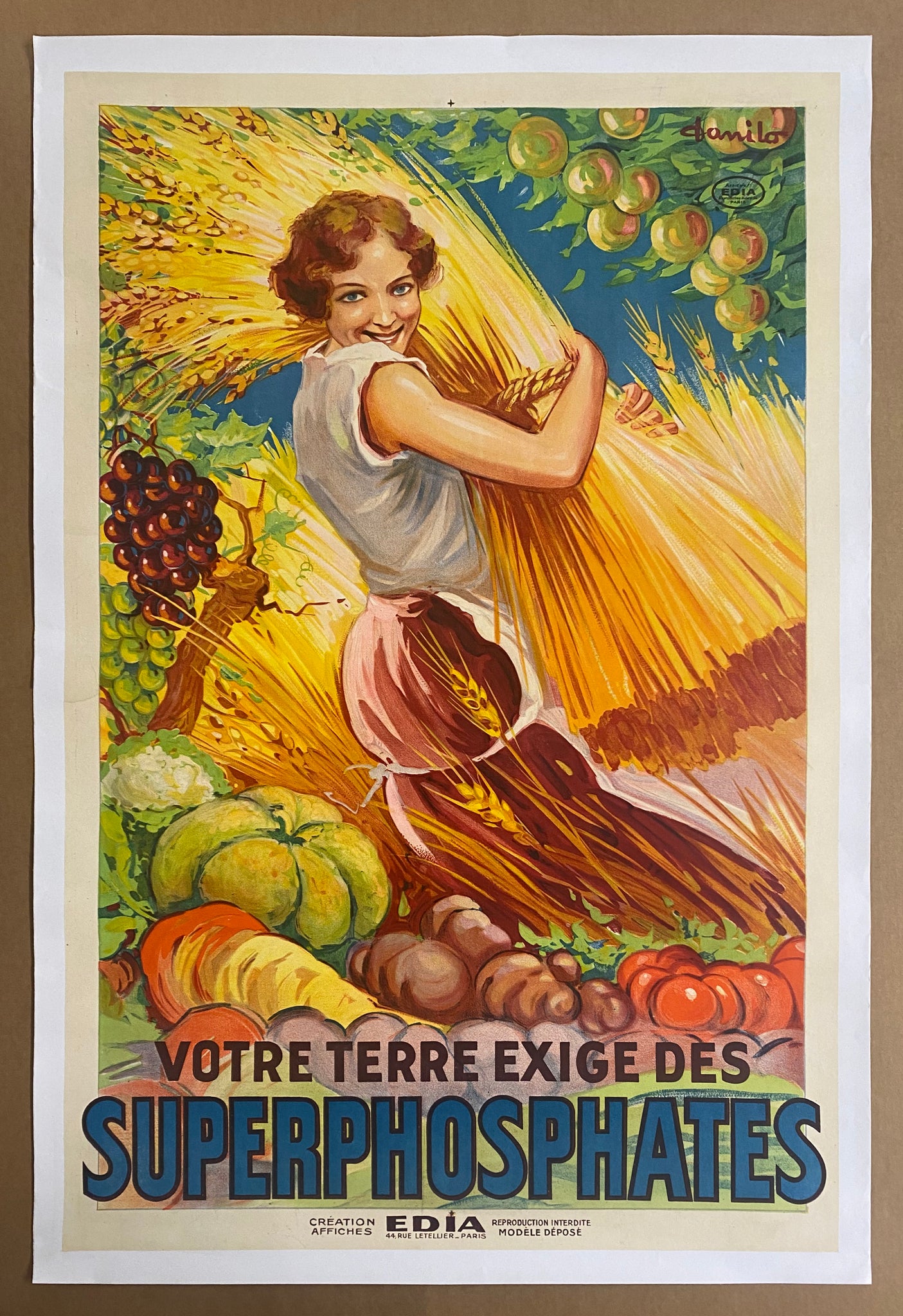This is a detailed vintage advertisement poster for plant garden fertilizer, framed with a white mat and tan mat border. The artwork, reminiscent of an oil painting, features a robust depiction of a woman with short red curly hair, standing and smiling. She is attired in a white sleeveless shirt, a long red skirt, and a white apron tied around her waist. She holds a large sheath of bundled wheat stalks with a rope tied in the middle. To her side and at her feet, a cornucopia of vibrant fruits and vegetables is displayed, including tomatoes, potatoes, green and purple grapes, a large cauliflower, a green gourd, and other produce. Behind her, a tree bearing green apples is visible, adding to the pastoral scene. The artist's signature can be found in small black letters in the top left corner of the poster. Below the main image, French text is centered, including "Votre Terra Exige" in black and "Super Phosphates" in bold blue letters with a black border, indicating the product being advertised. The overall aesthetic blends rich colors and agricultural abundance, capturing the essence of fruitful harvests.